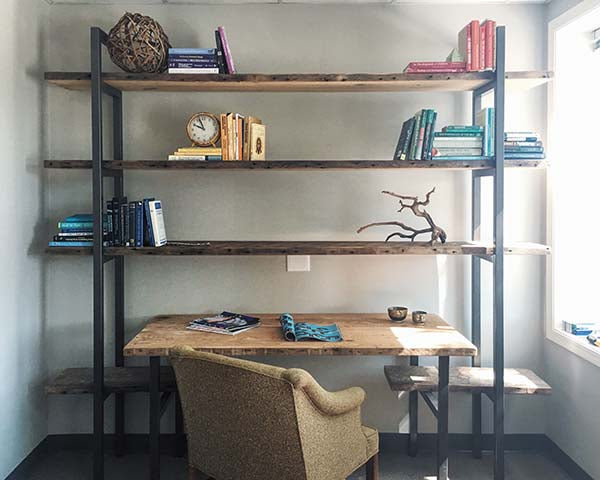This image portrays a cozy and well-organized small room featuring a multi-functional bookcase desk unit against a white wall. The bookcase consists of three high shelves and one low shelf, merging into a desk at the bottom, with a soft, cream-colored armchair stationed in front. The shelves are arranged with a mix of books and decor: the top shelf has casually stacked books and decorative items on the left, the middle shelf showcases an antique clock among grouped books, and the bottom shelf to the right contains both standing and laying down books alongside a tree sculpture. The desk surface has two or three magazines and a few small bowls. To the right of the bookcase, a window emits bright white light, illuminating sections of the shelving. The room is framed by black bars holding three tiered brown wooden planks, reinforcing the shelving structure and adding a touch of rustic elegance to the space.